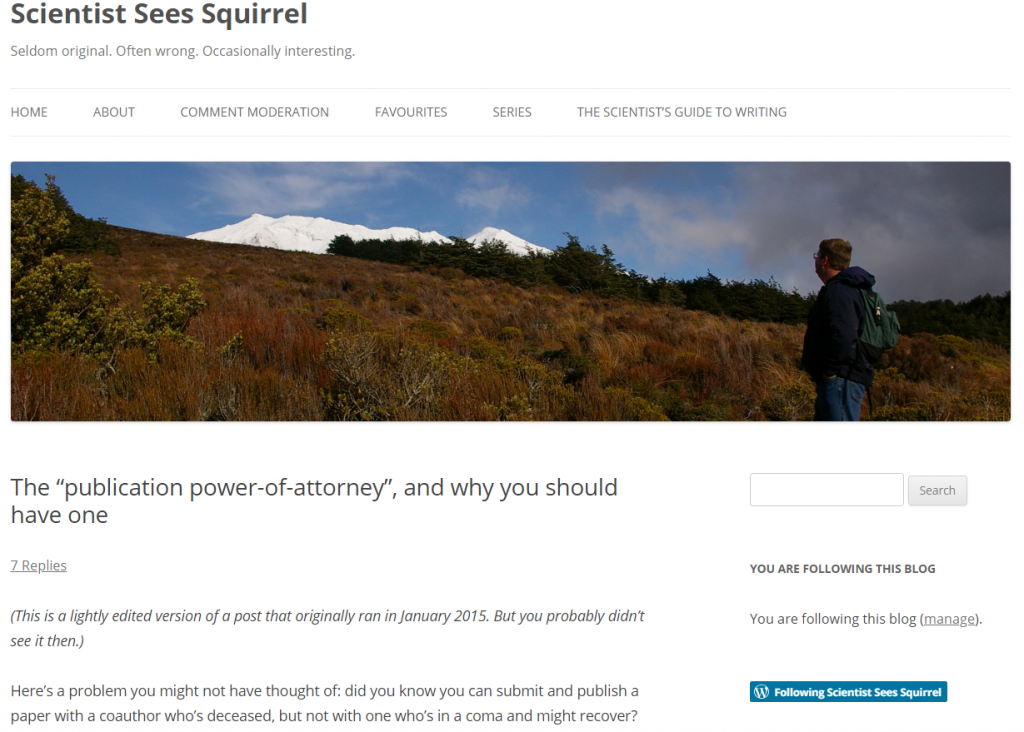A detailed caption for the cleaned-up image might read:

"This is a screenshot of a webpage titled 'Scientist Sees Squirrel,' with the tagline 'Seldom Original, Often Wrong, Occasionally Interesting' displayed in gray beneath the main title in black. The navigation bar at the top of the page features tabs labeled Home, About, Comment, Moderation, Favorites, Series, and The Scientist's Guide to Writing, all in gray. Below the tabs, a panoramic photograph captures a striking outdoor scene. The image prominently features a man dressed in a blue hoodie, jeans, and glasses, with blonde hair and a green backpack. His hands are in his pockets as he gazes thoughtfully at an ice-capped mountain under a serene blue sky dotted with clouds. The diverse hues of the grass around him range from orange and yellow to green. Beneath the photograph, the current article title reads 'The Publication Power of Attorney and Why You Should Have One.' Additionally, there is a search button and a blue button that says 'Following Scientist Sees Squirrel.'"